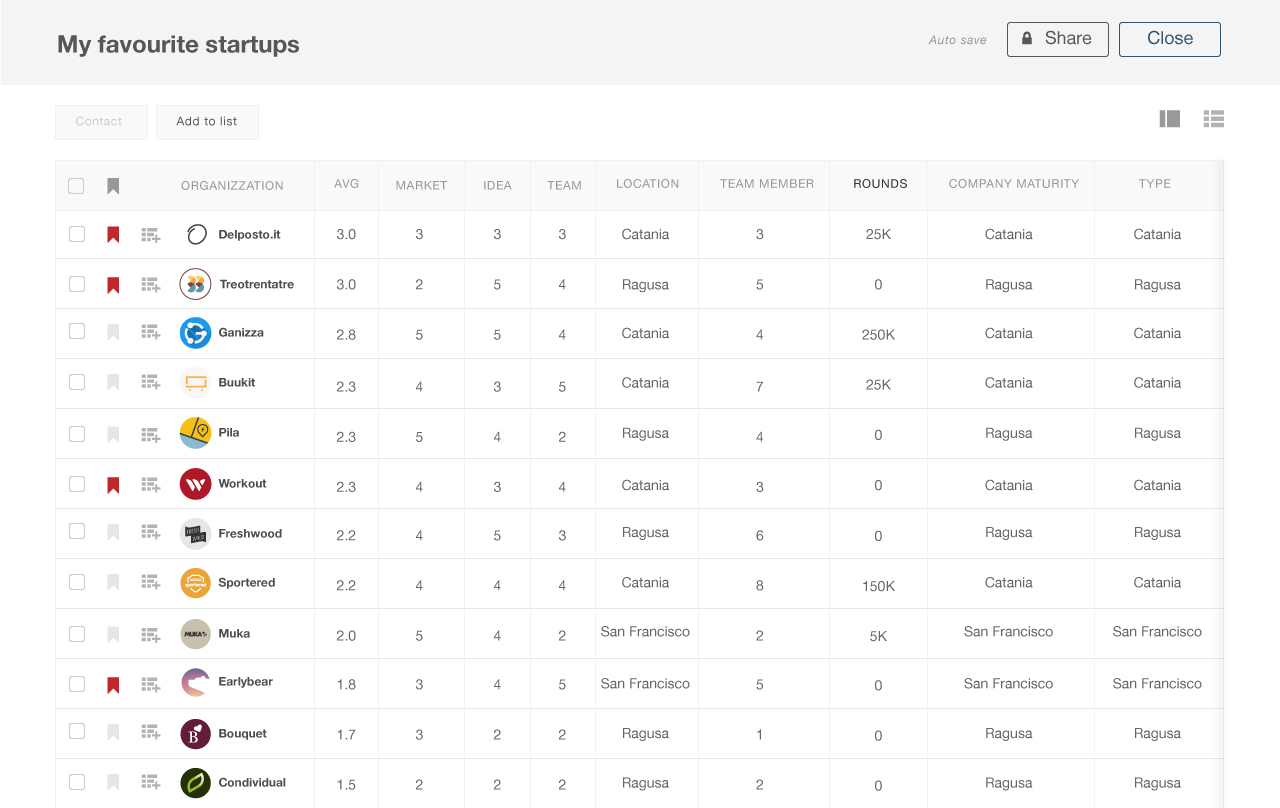In the "Websites" category, the webpage features a grey bar at the top labeled "My Favorite Startups," with an auto-save function. The bar includes a locked "Share" button and a "Closed" button. Below this, navigation options such as "Contact" and "Add to List" are available, along with a menu button.

The main content area displays a detailed list header with categories including "Organization," "Average," "Market," "Idea," "Team Location," "Team Members," "Rounds," "Company Maturity," and "Type." 

Four startups, marked with red flags to indicate they are saved, are listed with specific details:
1. **Del Posto** - Average score of 3.0, 25,000 rounds.
2. **Trio Trintarte** - Average score of 3, a team of 4 members, and zero rounds.
3. **Workout** - Zero rounds indicated.
4. **Early Bear** - Located in San Francisco, also has zero rounds.

Each entry provides a comprehensive look into the status and metrics of these startups, aiding in the evaluation and comparison of their potential.